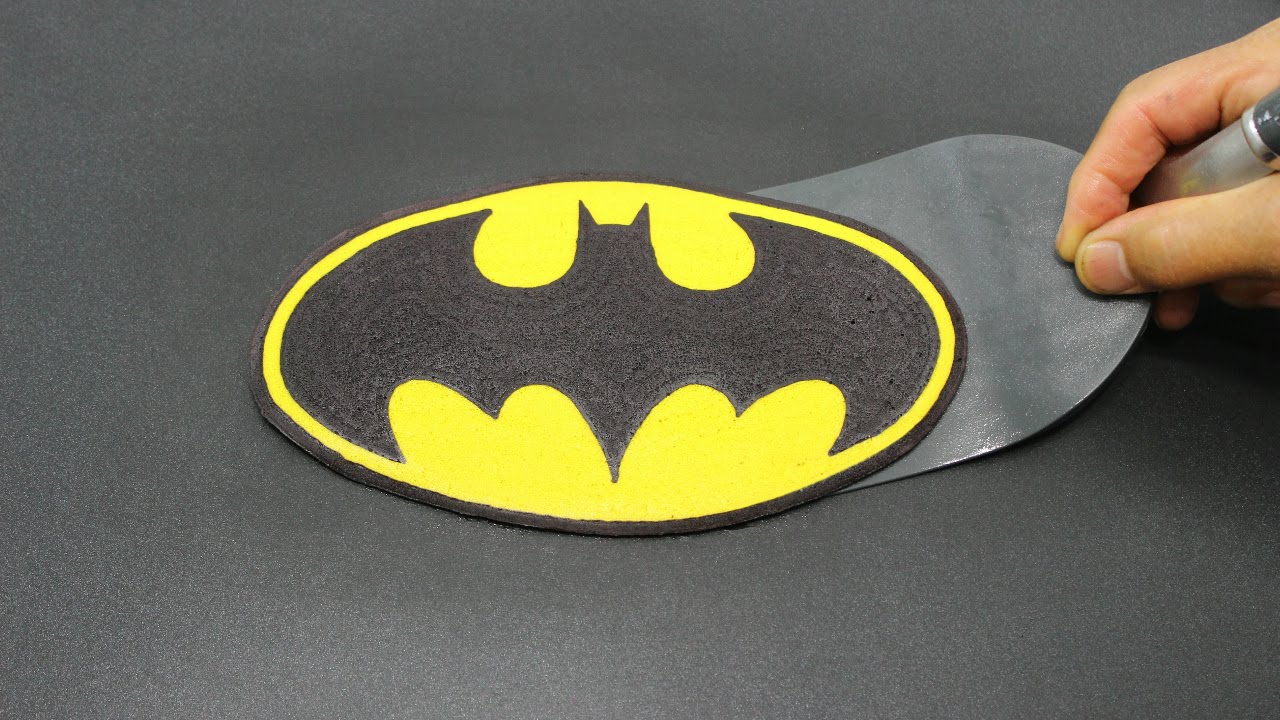In the image, a dark black or gray background contrasts against a white person's hand, which is positioned on the far right. The hand, featuring neatly trimmed nails and a silver ring on one finger, firmly grips a metal spatula with a black plastic handle. The spatula is in the process of peeling off a Batman logo sticker. The iconic logo, an oval shape encompassing a black bat on a yellow background, is central to the image. Subtle details, such as yellow flowers embellishing the logo and a round black sticker with a yellow trim, can be observed on the spatula. The scene captures the meticulous removal of the sticker from the surface, creating an intriguing visual focus on the hand's delicate yet precise action with the spatula.